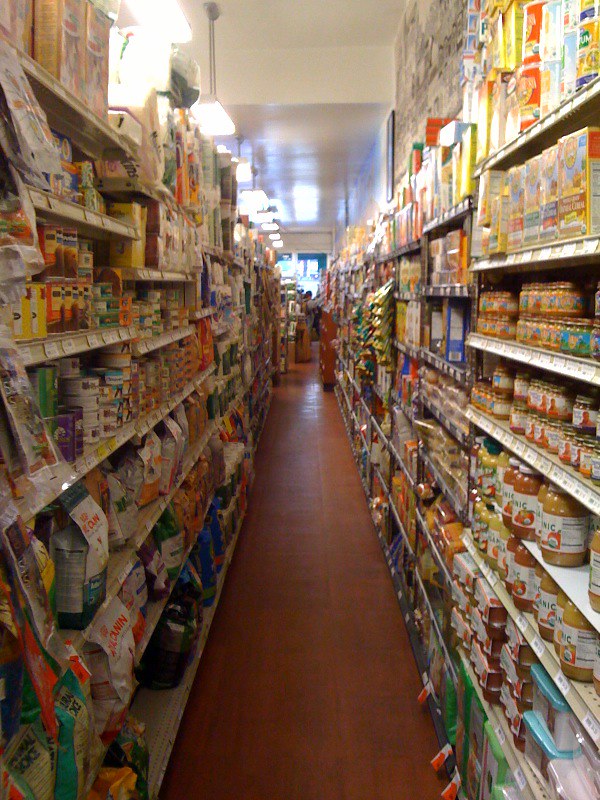The image is a detailed scene of a grocery store aisle, brightly lit with a white ceiling, showcasing a wide array of colorful products. The floor is a dark brown color. On the left side of the aisle, there are shelves stocked high with products, including cans featuring dog food and chow, labeled with animals like dogs and cows. Several bright, multicolored tags, though unreadable due to blurriness when zoomed in, suggest pricing details. The left side also features packages and treats hanging from plastic. On the right side, there's a variety of items like applesauce and baby food with jars and packaging in colors like yellow, orange, green, red, and purple. There are also larger jars likely containing applesauce and tubs at the bottom that are blue and clear. The aisle appears spacious and long, filled with a myriad of jars, cans, and packages.